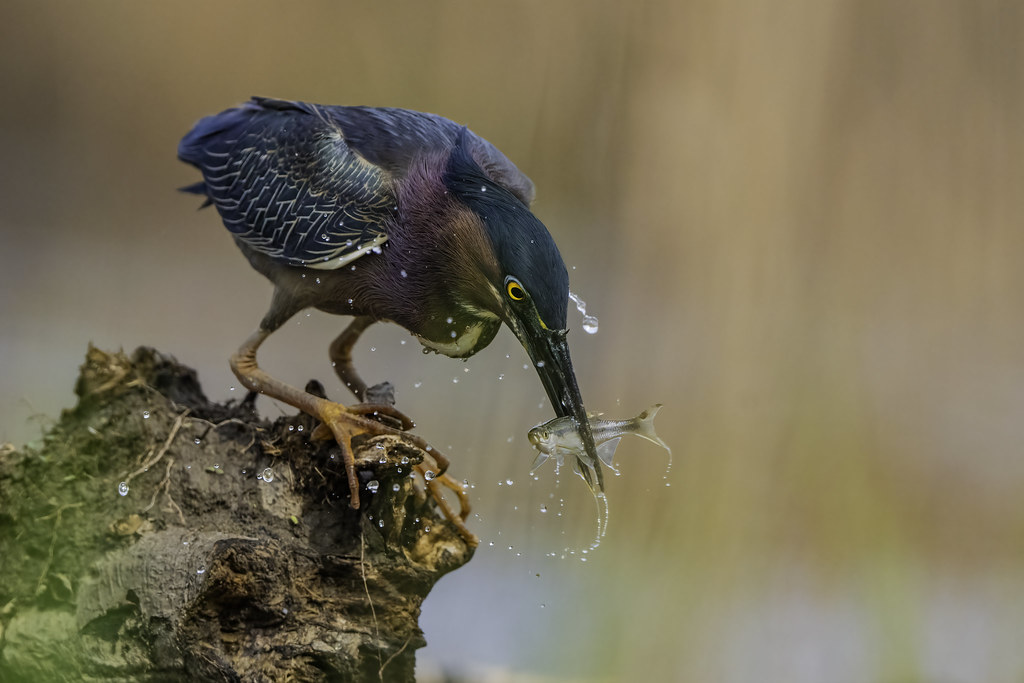In this photorealistic close-up image, a strikingly colorful seabird with a long beak is depicted catching a small fish slightly larger than a goldfish. Water droplets cascade from the bird's beak and the fish, hinting at the recent splash from the catch. The bird's vivid plumage showcases a brilliant mix of colors: a blue head, violet-mauve and pinkish-purple feathers around the neck, a blue and white back, and a brownish-green breast. Its orange eyes stand out vividly. Perched on a muddy, mossy outcropping resembling a beaver dam or old tree trunk, the bird's long legs are visible. The background is artistically blurred into muted tones of brown, pink, green, and blue, emphasizing the bird and creating an impression of an indistinct aquatic environment.